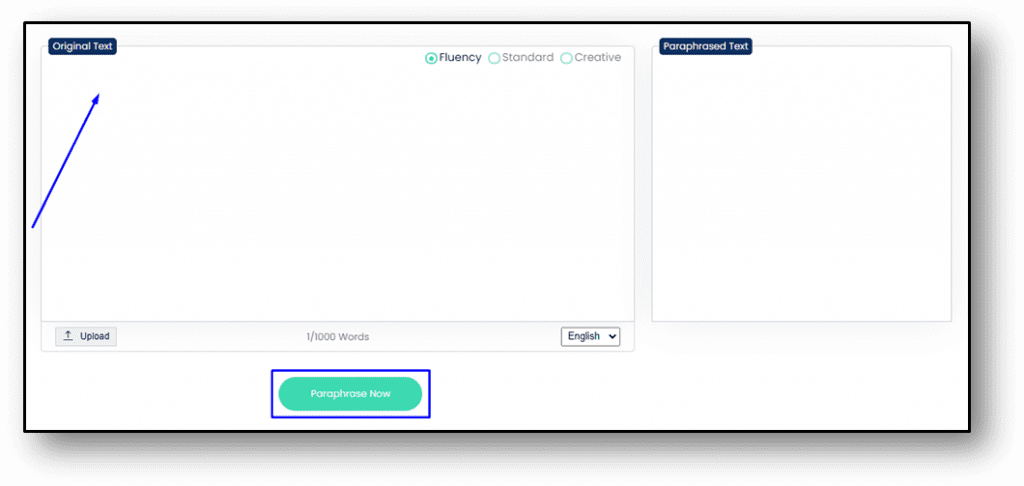This image displays a screenshot of a minimalist web application designed for text enhancement. The interface is characterized by a clean, white background and is organized into two principal sections within a long rectangular frame. 

On the left side, there is a larger rectangular text box labeled "Original Text," distinguished by a navy blue banner with white text. This section is indicated by an added blue arrow pointing towards it, suggestive of user interaction. At the upper right corner of this box, three selection options are available: "Fluency," "Standard," and "Creative," with the "Fluency" option currently selected.

Adjacent to the larger text box is a smaller square box on the right, which is labeled "Paraphrased Text" in the upper left corner. This area is designated for displaying the paraphrased output of the original content.

In the lower portion of the interface, a prominent green button labeled "Paraphrase Now" is positioned, emphasized by an added blue box meant to draw attention to its function.

Notably, both text boxes are currently blank, indicating the application is ready for user input and subsequent processing.